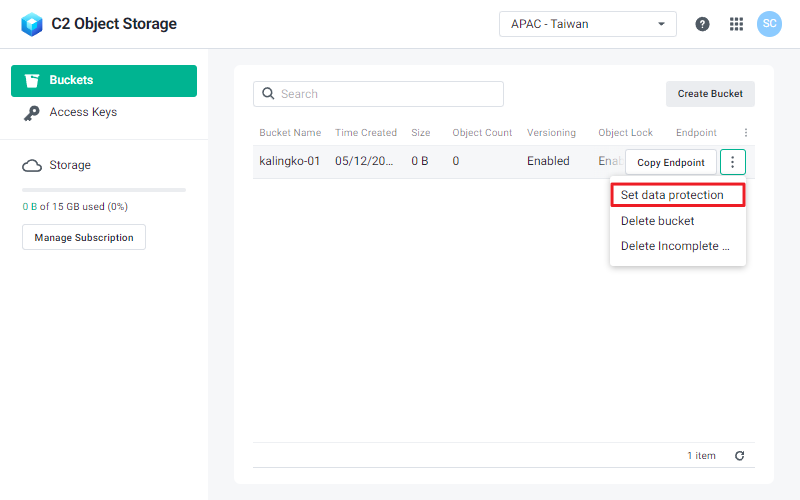Displayed on the page, on the left side, is a section featuring a stylized capital "C" followed by the number "2" under the label "Object Storage." The symbol preceding the capital "C" is designed to appear three-dimensional, with light and dark blue shading and a white diamond shape in the center to enhance the three-dimensional effect. The currently selected region from the drop-down menu is "APAC Taiwan." To the far right, the logged-in user appears to be identified by the initials "SC."

Below this, the page features a green navigation bar with options labeled "Buckets," "Access Keys," and "Storage." The "Buckets" option is currently active. There is also an option labeled "Manage Subscription." To the right, there is a separate area containing an additional search bar and a "Create Bucket" button. This section details information columns titled "Bucket Name," "Time Created," "Size," "Object Count," "Versioning," "Object Lock," and "End Point."

Under the "Copy End Point" section, options include setting data, deleting the bucket, or deleting incomplete tasks. The "Set Data" option is highlighted with a red border.